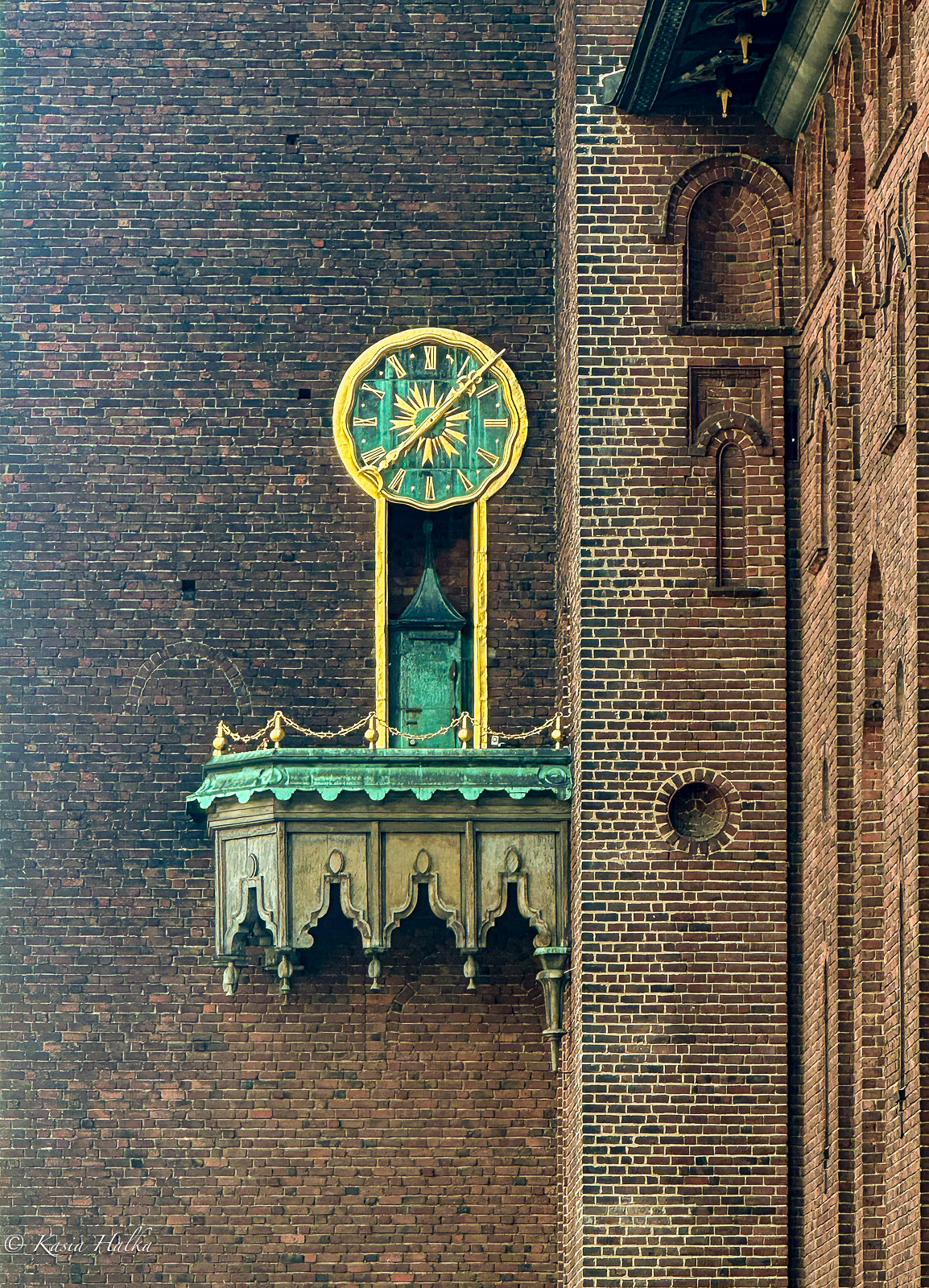A stunning image captures a grandiose, aged red brick building dominated by an intricate green and gold clock. The clock, featuring Roman numerals, is richly adorned and commands attention as its large hands point between the 1 and 2, and the 7 and 8. Below the clock, an arched green door provides entry to the towering structure, its facade weathered and blackened in places, adding a sense of historical depth. To the left, a series of arches contribute to the architectural complexity, while a balcony adorned with a golden chain barrier adds an opulent touch. The building's exterior reveals a striking green patina, blending harmoniously with the luxurious elements and the overall grandeur of the scene.